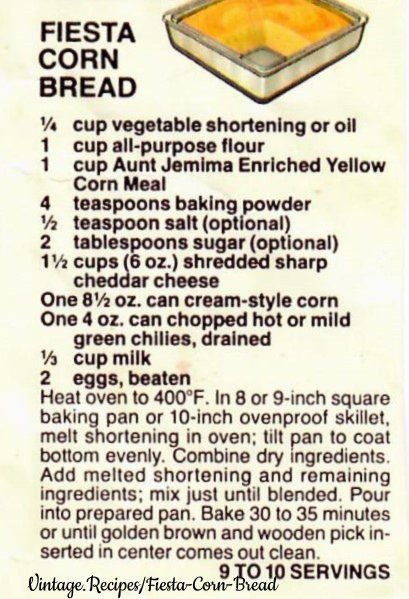This image, likely a scanned recipe page, depicts a vintage Fiesta Cornbread recipe from the website "Vintage.Recipes.Fiesta.Corn.Bread" as indicated by a watermark at the bottom. The image shows a slightly yellowed, color scan with black text on an off-white or light gray background. At the top left is the recipe title "Fiesta Cornbread" along with a drawing of a square baking dish filled with cornbread, missing one piece to reveal its texture. The recipe caption lists detailed ingredients including:

- 1 1⁄4 cup vegetable shortening or oil
- 1 cup all-purpose flour
- 1 cup Aunt Jemima enriched yellow cornmeal
- 4 teaspoons baking powder
- 1⁄2 teaspoon salt
- 2 tablespoons sugar
- 1 1⁄2 cups shredded sharp cheddar cheese
- 1 8 1⁄2-ounce can cream-style corn
- 1 4-ounce can chopped hot or mild green chilies, drained
- 1⁄3 cup milk
- 2 eggs, beaten

The instructions for baking are also provided, making enough cornbread to serve 9-10 people. The overall appearance suggests that it has been re-shared multiple times, contributing to its low quality.